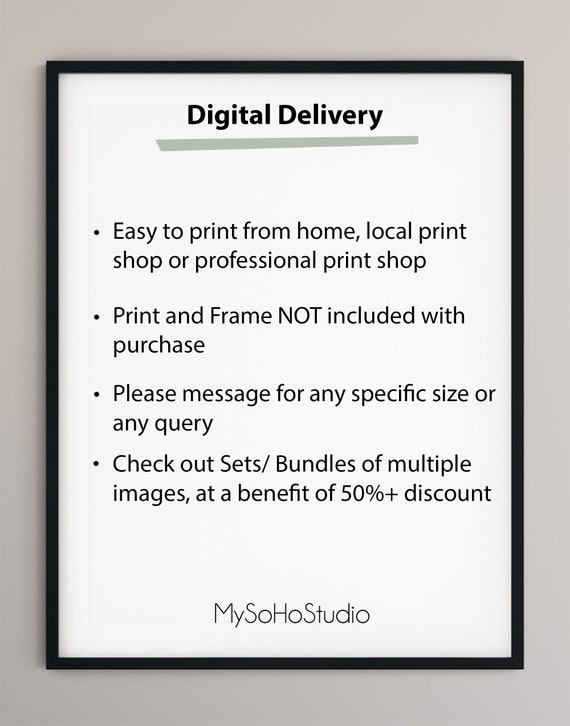This grayscale black and white image is an advertisement featuring a black frame against a light-colored background. Inside the frame, the bold text "Digital Delivery" is prominently displayed at the top. Below this title are four bullet points detailing the services offered: "Easy to print from home, local print shop, or professional print shop", "Print and frame not included with purchase", "Please message for any specific size or any query", and "Check out sets/bundles of multiple images at a benefit of 50% plus discount." The text concludes with "My Soho Studio" at the bottom. The overall message conveys that My Soho Studio offers various digital delivery options for their print products, emphasizing ease of printing, customer service, and significant discounts on bundled sets.